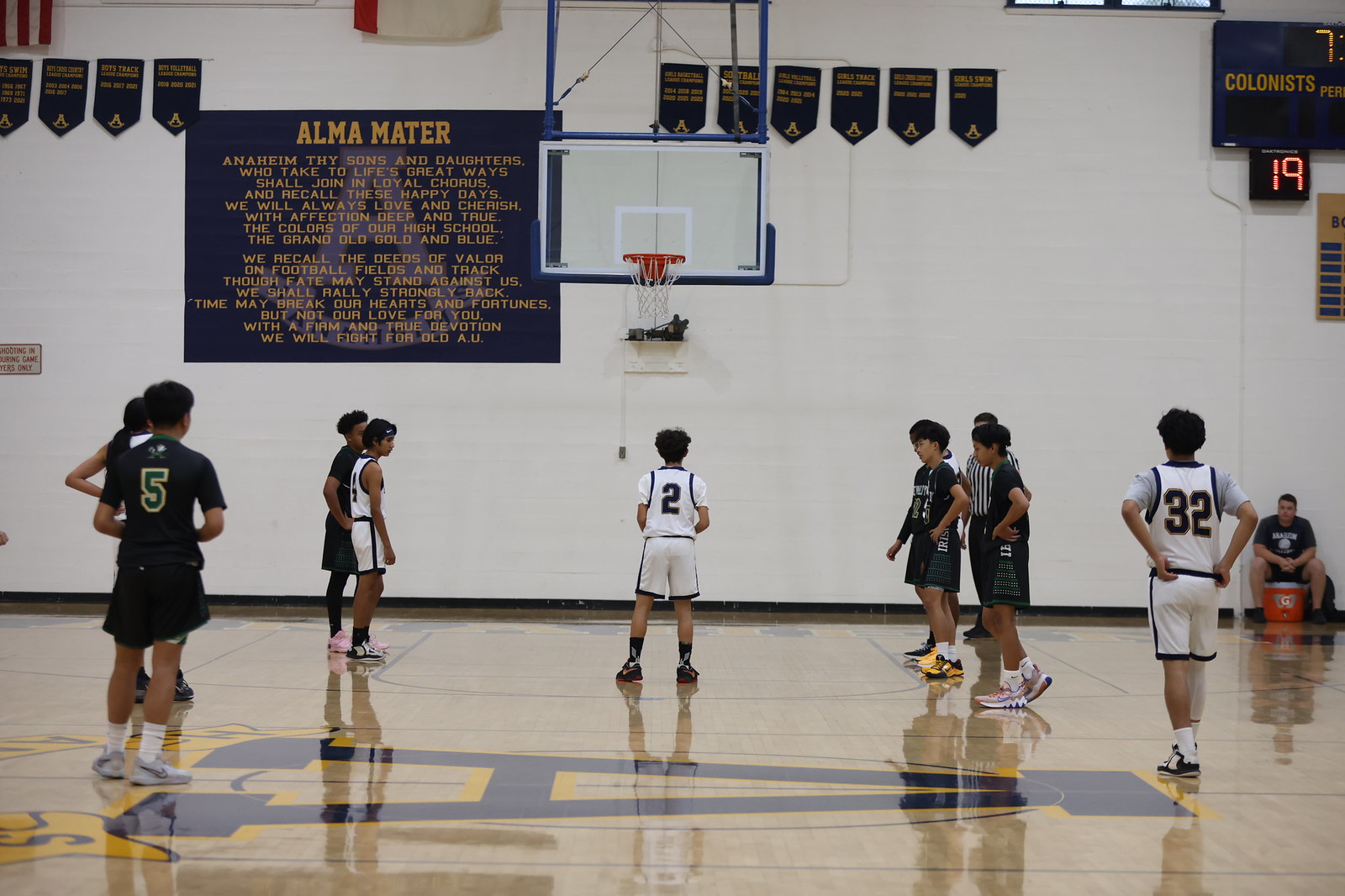The photograph captures a dynamic scene of a high school basketball game taking place in a school gymnasium. The gym's white wall prominently displays a plaque labeled "Alma Mater" with various championship banners hanging above it, indicating the team's past achievements. The court features a shiny brown hardwood floor with a large "A" logo painted at its center, suggesting the school's name begins with the letter A, possibly Anaheim. In the center of the image, a player in a white jersey, numbered two, is about to shoot a free throw while the opposing team, dressed in black jerseys, stands at the free throw line. The clock shows 19 seconds with about seven minutes left in the game. Observant details include a person seated on a Gatorade bucket in the bottom corner, adding a touch of the sidelines' typical hustle. The scene vividly depicts the intensity and community spirit of high school sports.